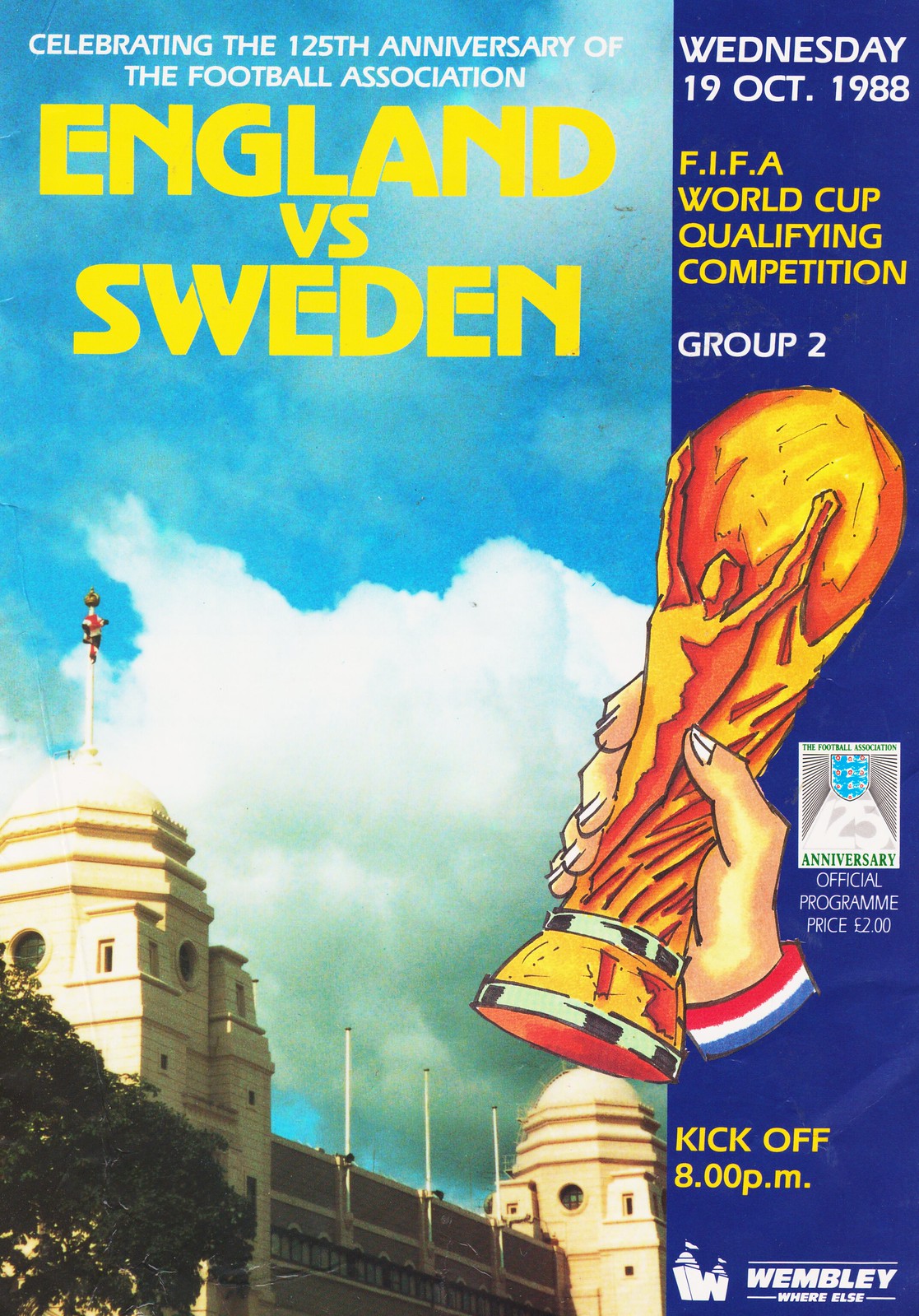This tall, rectangular image appears to be the front page of a sports program from October 19, 1988, commemorating the 125th anniversary of the Football Association. The majority of the image is dominated by a photograph of a bright blue sky with a substantial, thick cloud that transitions from white at the top to greener and grayer at the bottom. Below the cloud, an off-white and gold building with a large dome on the left side and a green tree in front is depicted at an angle. 

On the top part of the image, in white, all capital letters, it reads "CELEBRATING THE 125TH ANNIVERSARY OF THE FOOTBALL ASSOCIATION," and below that, in bold yellow capital letters, "ENGLAND VS. SWEDEN." A vertical blue rectangle on the right side contains additional text: "Wednesday, 19 October 1988" and "FIFA World Cup Qualifying Competition Group Two" in yellow text, along with a drawing of a hand holding what appears to be the FIFA World Cup trophy. At the bottom right corner, it states "Wembley Where Else" in white, likely indicating the venue or the logo of the publication, and the kickoff time is noted as "8 PM." The program's price, two pounds, is also mentioned in this section.